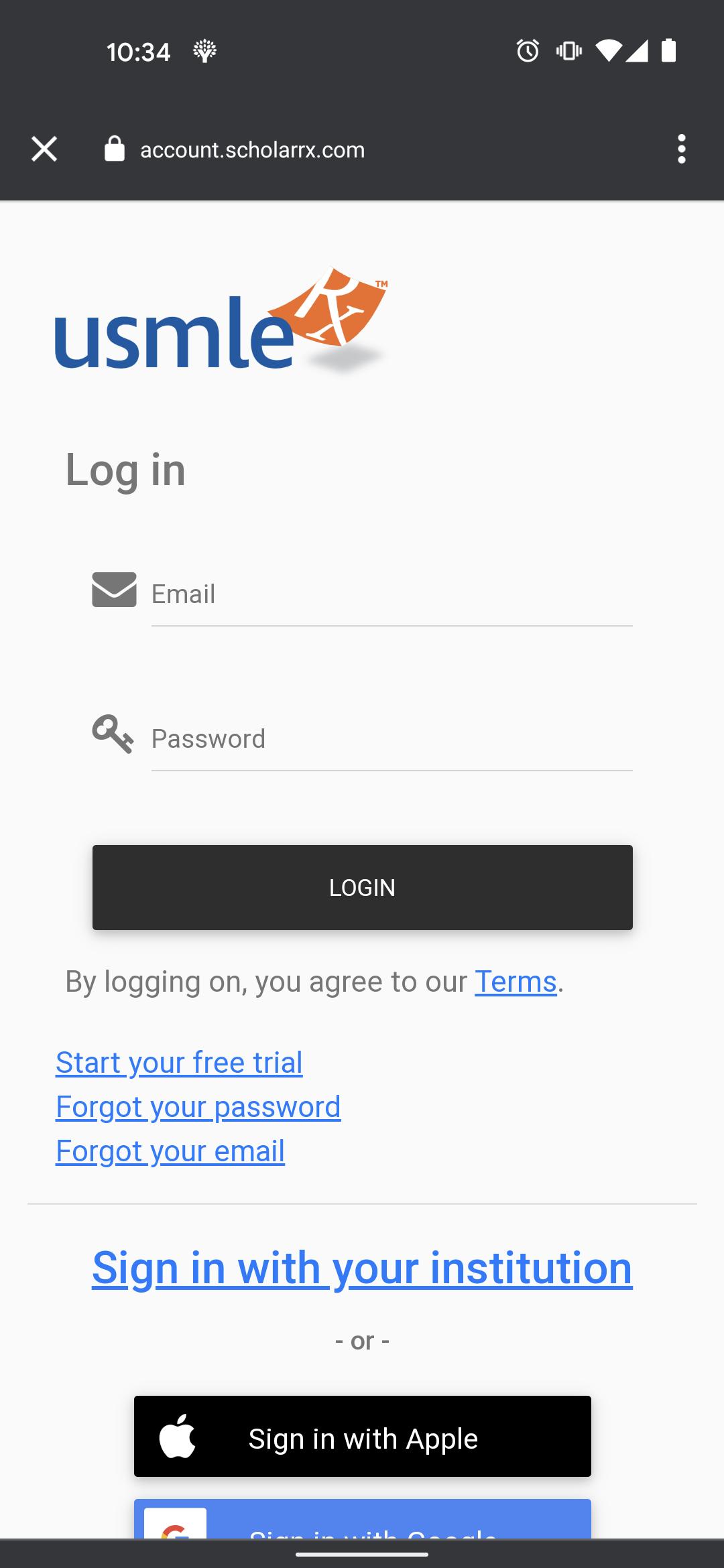The screenshot image features a detailed user interface of a login page for ScholarRx, a medical education platform. 

At the very top of the screen, there's a black banner. On the left side, the time reads 10:34. Further to the right, several icons are visible: an alarm clock icon, a phone rotation icon, a silence notification icon, a fully lit Wi-Fi signal icon, and a fully charged battery icon. 

Below this, still within the black banner, a white "X" is displayed in the lower left-hand corner, followed by a lock icon and the text "accountscholarrx.com," indicating it is a secure page.

Beneath the black banner, there is blue text that reads "USMLE" (United States Medical Licensing Examination), alongside an orange square with the letters "RX," symbolizing "prescription."

Scrolling down, there is a login section. The word "LOGIN" is prominently displayed, followed by input fields for the email address and password. Below the password field, a black button centered within the interface reads "Login."

An additional line of text beneath the login button indicates that by logging in, users are agreeing to the terms and conditions associated with the platform.